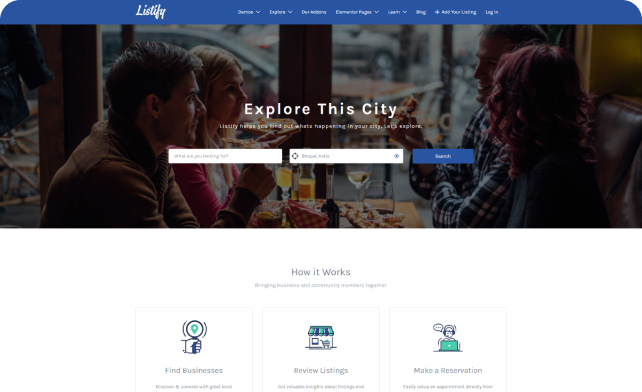**Caption:** 

The image is a screenshot of a website's home page, prominently featuring a dark blue banner at the top that reads "Listify." This banner includes several navigation categories such as "Explore" and "Blog," along with a "Login" section towards the right side. Below the banner, the background image displays a lively scene of four people sitting at a table, enjoying a meal together. The central text overlay on this image invites users to "Explore This City." Positioned beneath this message are two search bars aligned horizontally, and on the far right end of these bars is a "Search" button, indicating where users can input and submit their queries.